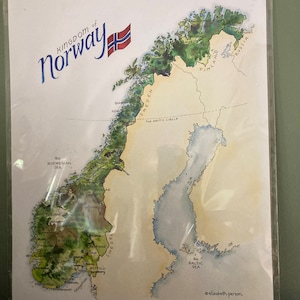This image depicts a highly detailed postcard of Norway, still encased in a clear protective sleeve. Dominating the upper left corner is the bold, blue phrase "Kingdom of Norway" in an elegant, italicized cursive font. Adjacent to it is the iconic red and blue flag of Norway, slightly jagged in its representation but unmistakably accurate. The right side of the postcard features a meticulously drawn map of Norway, outlined prominently in green to emphasize its geographical shape. The map includes light pastel yellow borders delineating neighboring countries, with labels identifying key locations and cities. The background of the postcard is white, enhancing the overall clarity of the depicted features. This vibrant illustration is displayed against a green wall, adding a final touch of contrast.